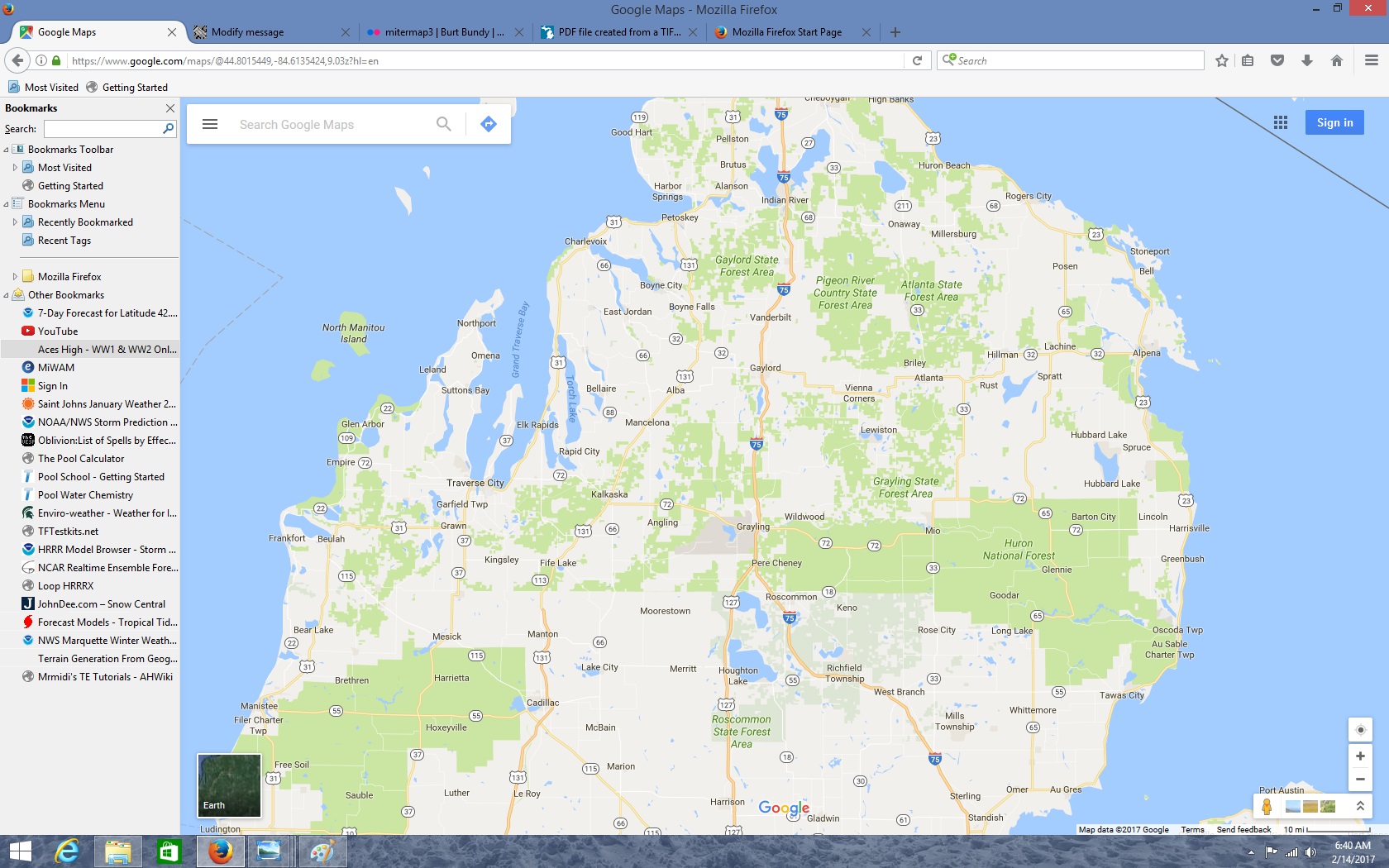A detailed Google Maps interface is displayed within the Mozilla Firefox browser on a desktop screen. At the top, a light blue strip marks the browser's tab section, with numerous open tabs visible. An open bookmarks bar showcases various bookmarked sites, including a Microsoft sign-in page and several other unnamed URLs. The main map area features a large land region with an off-white background interspersed with green patches representing different types of greenery or recreational areas.

The map is peppered with extensive black text labels denoting places, streets, and landmarks. Distinct orange lines depict highways, while blue, red, and white numbered markers indicate specific routes and interstates. Areas covered by water are illustrated with a light blue background. A blue sign-in square is notable at the upper portion of the image, inviting user authentication. Additionally, several icons line the bottom of the screen, emblematic of various functions and tools available within the Google Maps interface.